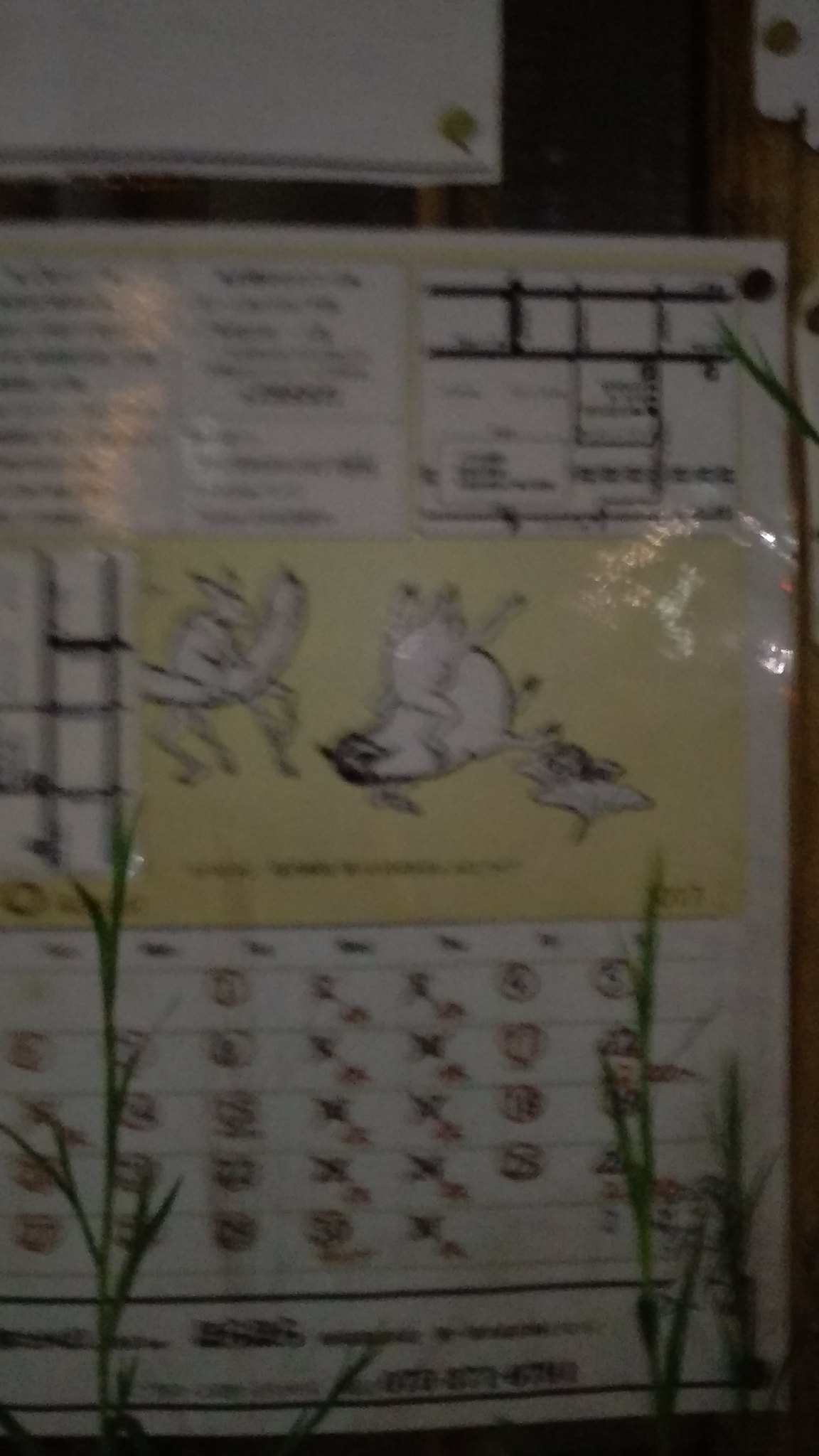The image is somewhat indistinct due to a significant blur, making the finer details challenging to discern. However, visible elements suggest it depicts a dark wood bulletin board, possibly located in a home or store. 

The board prominently displays a laminated piece of paper, secured with black tacks. Positioned above this is a partially visible corner of another white piece of paper, affixed with a yellow tack. The main laminated document includes a small calendar at the bottom, featuring marked and circled dates.

The central portion of this paper presents a yellow rectangle adorned with clip art, although the exact nature of these graphics is unclear—potentially depicting animals or other ambiguous shapes. In the upper third of the paper, the right-hand corner possibly contains a map, while the left-hand corner includes text, both of which are unreadable due to the blur.

In the foreground, originating from the bottom edge of the image on both the left and right sides, appear three green plant stems or branches, further adding to the composition.